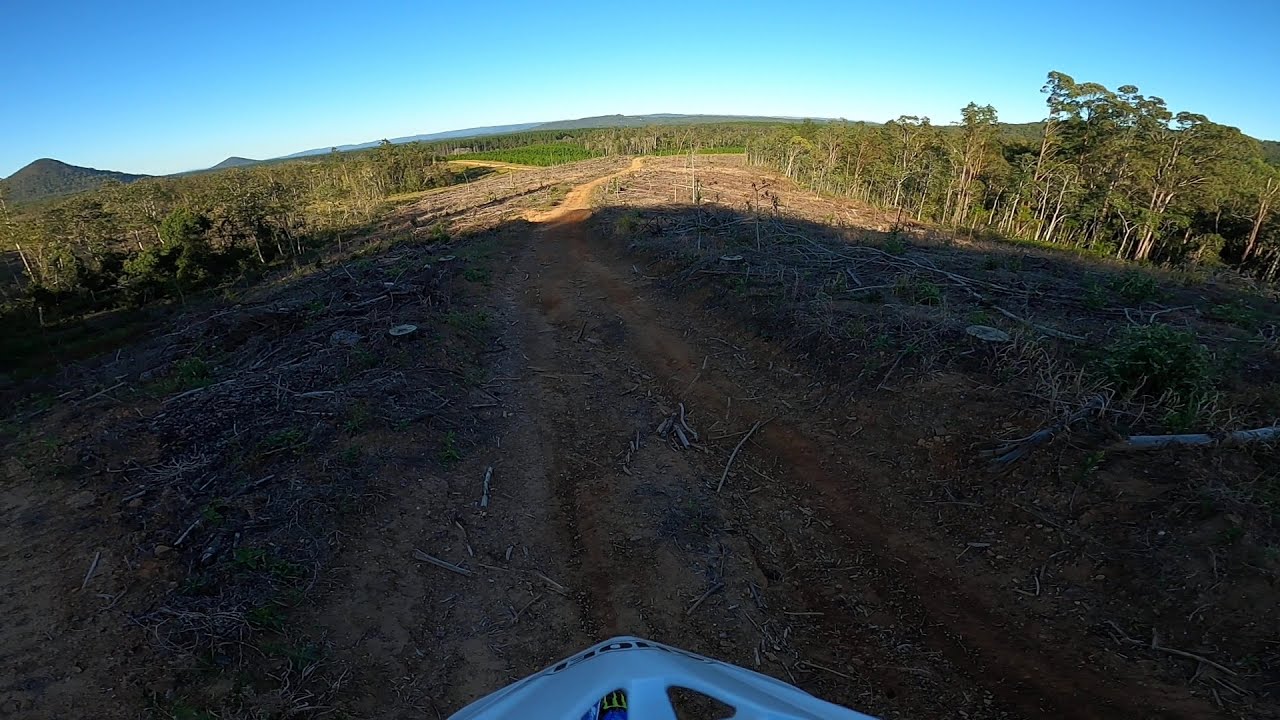This is a wide rectangular photograph of a narrow, unmetalled pathway winding through an outdoor setting. The pathway, composed of brown soil and light brown sticks, starts at the bottom of the image and stretches towards the center, eventually disappearing into the distance. On both sides of the road, there are patches of green and dried grass, with occasional tree limbs scattered around. The sides of the pathway are flanked by a mix of green, leafy trees, creating a forested backdrop. In the background, particularly on the left, there are rolling hills. Above, the sky is a clear, vibrant blue, illuminated by sunlight, indicating a sunny day. At the bottom of the picture, there is a metallic white, dome-shaped object, likely the front of a vehicle such as a bike, partially visible and adding a sense of presence in the foreground. The overall scene is characterized by a peaceful blend of natural elements under a clear sky, with shadows cast over parts of the pathway and surrounding grass, enhancing the depth of the image.